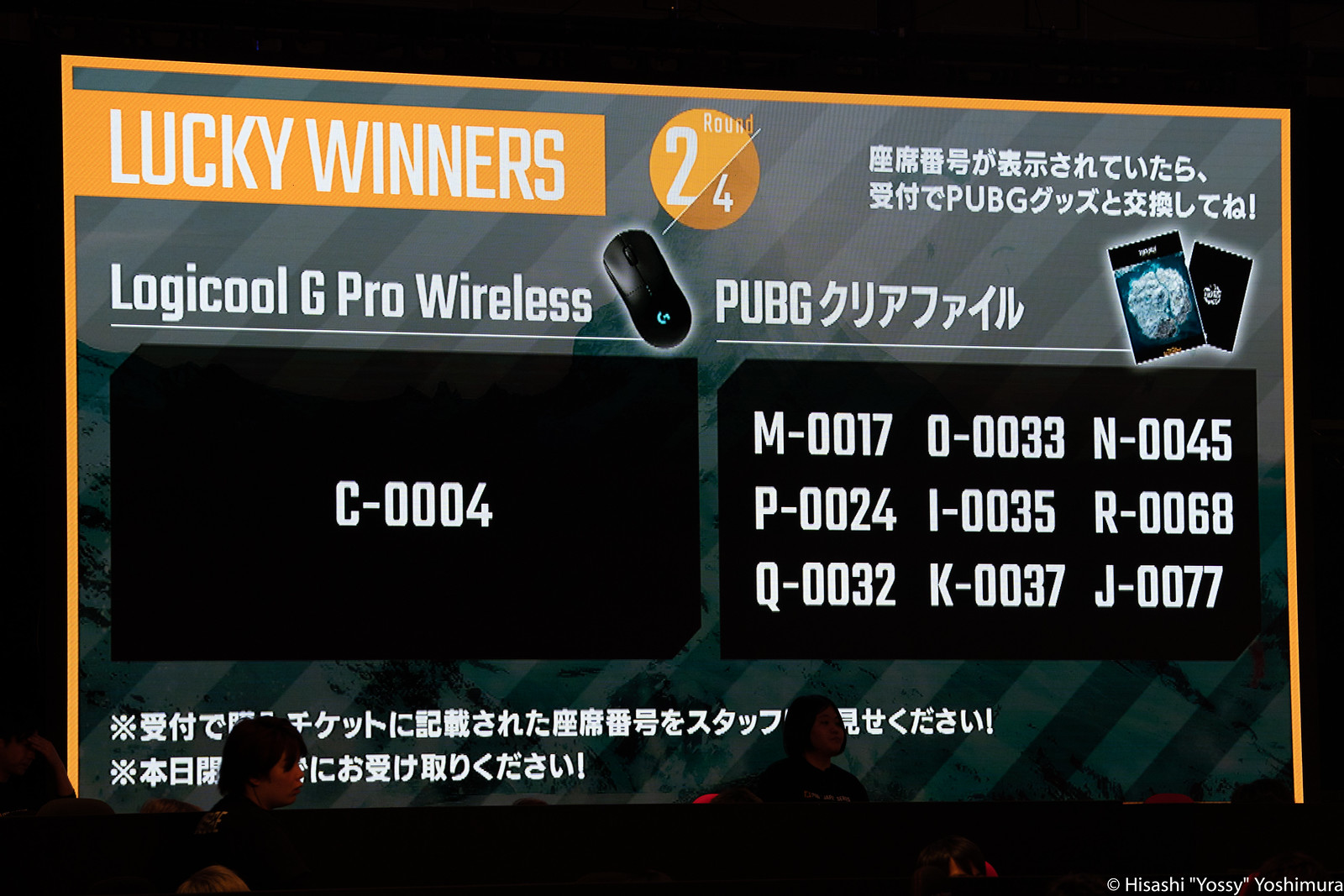The image displays a large, computer-generated screen projected in a theater or presentation room, evidenced by the visible heads of audience members at the bottom of the image. The top of the screen features a rectangular orange strip extending from the left edge, displaying the text "Lucky Winners" in white letters. Directly beneath this, the text reads "Round 2 of 4," with the number "2" inside a circle and a diagonal line between "2" and "4." To the right of this are characters in what appears to be an Asian language, possibly Chinese or Japanese.

In the middle section of the screen, to the left, the text "Logicool G Pro Wireless" is shown alongside an image of a computer mouse. Adjacent to this, on the right, is the word "PUBG" accompanied by additional non-English characters. Below this section, there are two rectangular black boxes. The box on the left contains the code "C-0004," while the box on the right displays a series of similar codes, each consisting of a letter followed by four numbers starting with double zeros.

At the very bottom of the screen, there's a string of additional characters in an Asian script, formatted in two rows. The name "Hisashi Yossi Yoshimura" appears in the lower right corner. Multiple audience members partially obstruct the bottom part of the screen, reinforcing the setting's immersive and large-scale projection.